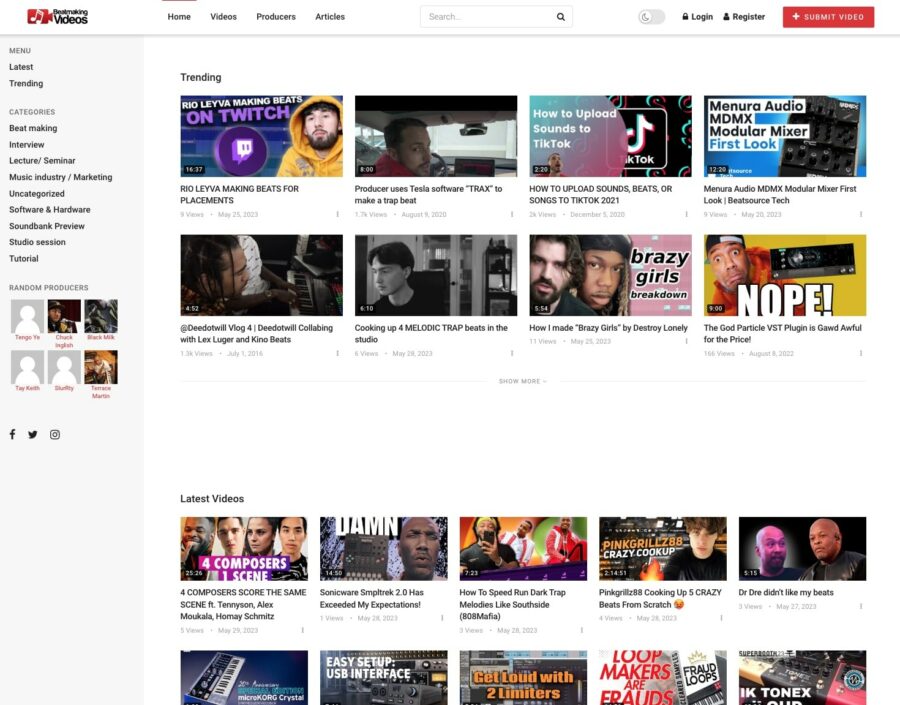In the top left corner of the image, there is a red box labeled "videos." Beside the box, a section entitled "Trending" is visible, suggesting this image is from YouTube. The upper part of the screen features two rows of video thumbnails, each displaying four clips or pictures. 

One thumbnail features a man wearing a yellow rain jacket with the caption "on Twitch." Another thumbnail further down and in black and white is labeled "Cooking up a melodic trap beat in the studio." On the far right, a thumbnail shows a man with a worried expression; the text on this image reads "NOPE!" with an exclamation mark, and it includes an image of a stereo with the caption "The good particle vest plug-in."

Below these thumbnails, there are two additional informational sections titled "Latest videos." One thumbnail within this section shows a person wearing a black shirt and sporting brown hair, with a fire emoji in the background, and is labeled "A Composer's Score." Next to it is an image of Dr. Dre, and to the left, a person illuminated in pink light with the caption "Dr. Dre didn’t like my beats."